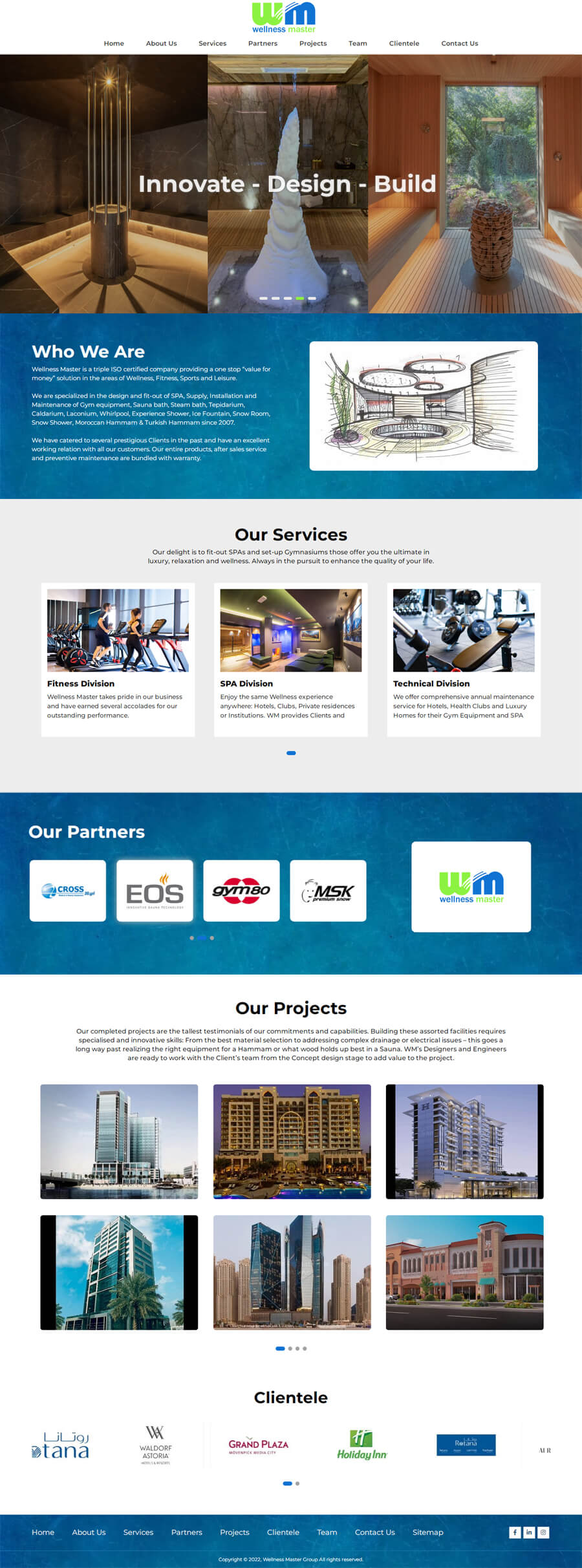This is a detailed description of a website layout. 

At the very top center, there is a logo with the letters "WM" where the "W" is green and the "M" is blue. Below the logo, there are small, unreadable black text options. Underneath this menu, there are three images showing different designs or construction projects. Above these images, in large white text, are the words "Innovate, Design, Build." Following this, there is a blue box containing large white text that reads "Who Are We." Inside this box, there are three paragraphs of white text which are not legible, accompanied by a hand-drawn architectural illustration.

Further down, in black text, the section titled "Our Services" is introduced. Below this heading, there are three images, each paired with a small paragraph of information.

Continuing further, a section titled "Our Partners" features four partner logos, followed by the "WM" logo once again. Below the logo, in black text, is a section labeled "Our Projects," accompanied by a descriptive paragraph in black text. This section includes six images depicting various cityscapes. Finally, at the bottom of the page, there is a section titled "Clientele" in black text.